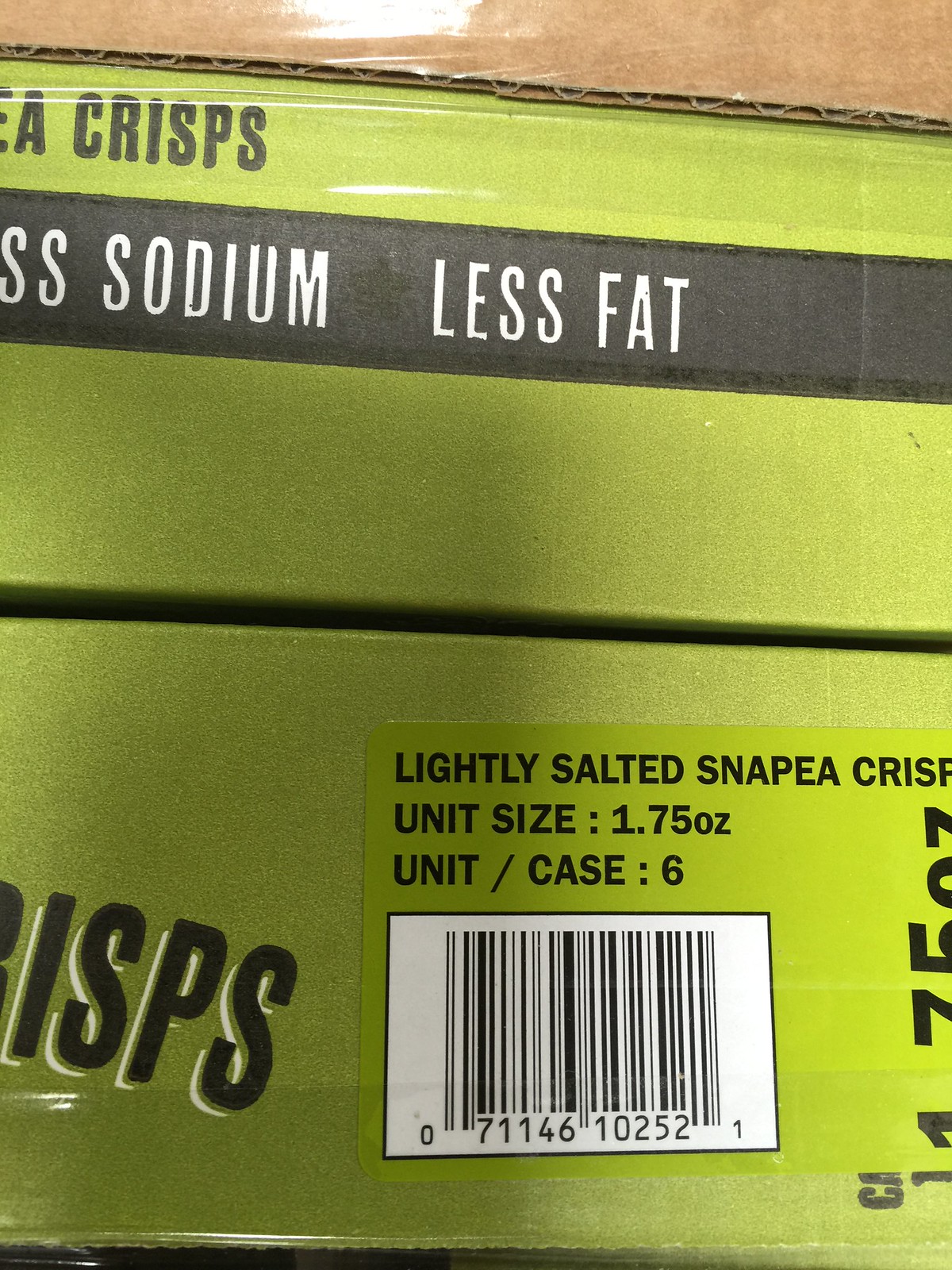The image showcases the edge of a retail box packaging for "Lightly Salted Snapea Crisps." The box features a prominent barcode and the nutritional highlights "Less Sodium" and "Less Fat" prominently displayed. The packaging is predominantly green, consistent with the branding of the Snapea Crisps. Additionally, various horizontal numbers are visible on the right-hand side of the box. The top part of the image reveals another cardboard box, suggesting that these are individual packs that are either awaiting shelf placement or part of a multipack. Overall, the image focuses on the details of the Snapea Crisps packaging within a larger cardboard container.